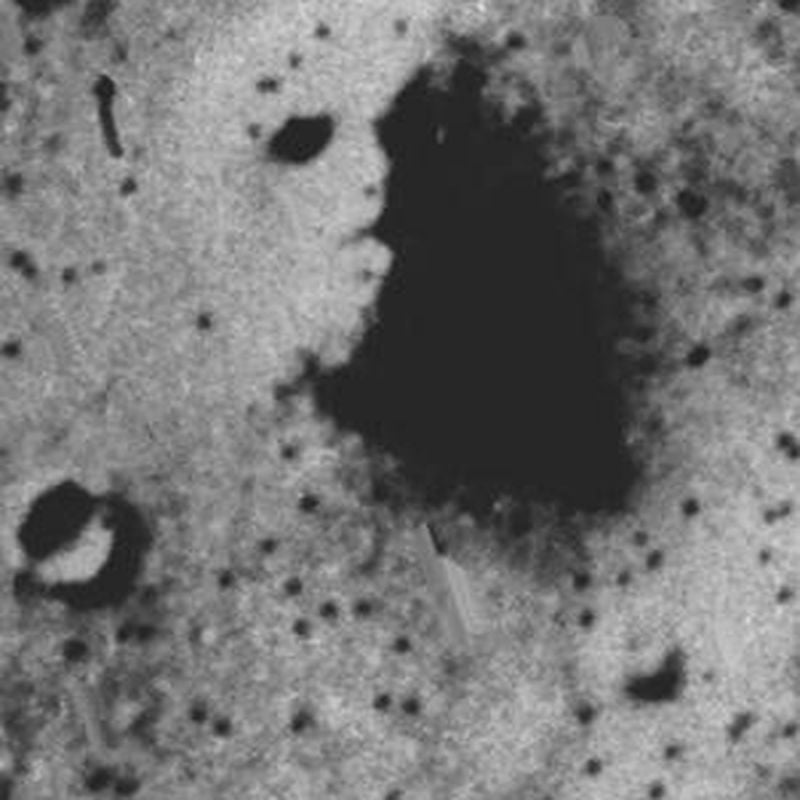The image is a grainy, black-and-white close-up that evokes the impression of a microscopic slide or an outdoor terrain, such as a moonscape or cave. Dominating the center of the image is a large, ominous-looking black splotch or crevice, surrounded by a light gray and white textured surface filled with numerous tiny black spots. The standout feature of this stark landscape is an uncanny outline within the black splotch, which resembles a human face gazing to the right, casting a significant shadow. This eerie visage—merely a coincidental pattern in the grainy photo—adds an otherworldly and surreal quality to the scene, reminiscent of the infamous man-in-the-moon image taken from above a desolate, lifeless terrain. The overall effect is detailed yet ambiguous, bridging the realms of microscopic and extraterrestrial landscapes.